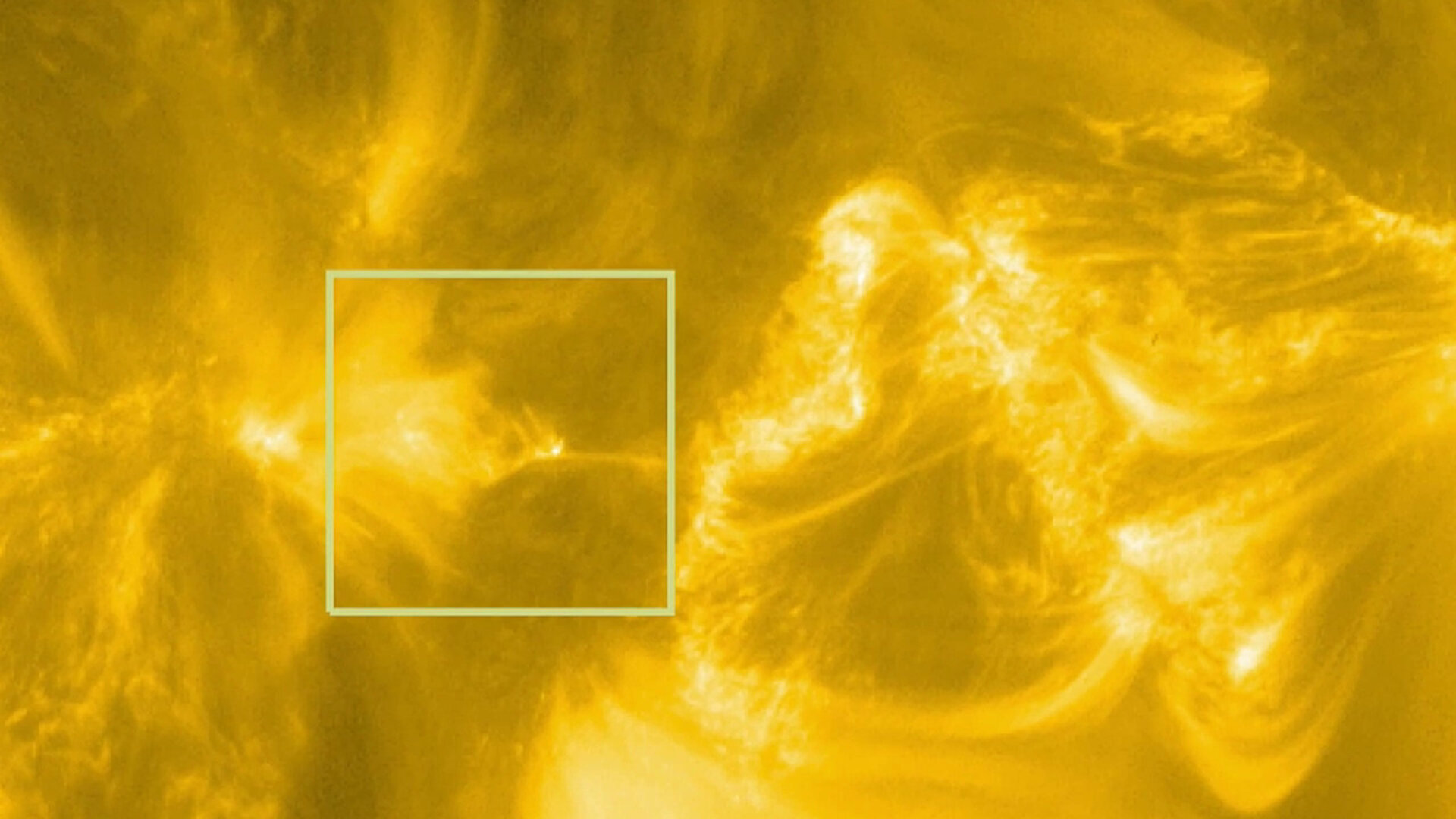This image predominantly features billowing flames and gas, likely from a star, possibly resembling our Sun. The scene is filled with swirling shapes of color that strongly resemble fiery solar flares. The color palette primarily consists of white-hot regions transitioning to vibrant oranges, dark golds, and even brown hues, all suggesting intense heat. The largest flame emerges from the right side, while a possible epicenter on the left is marked by a light green square, intended to draw attention to a specific area, although the exact focus remains unclear. The image, rectangular and somewhat hazy, lacks any textual annotations, contributing to an air of ambiguity about what specific detail is meant to be highlighted within the green-outlined area.